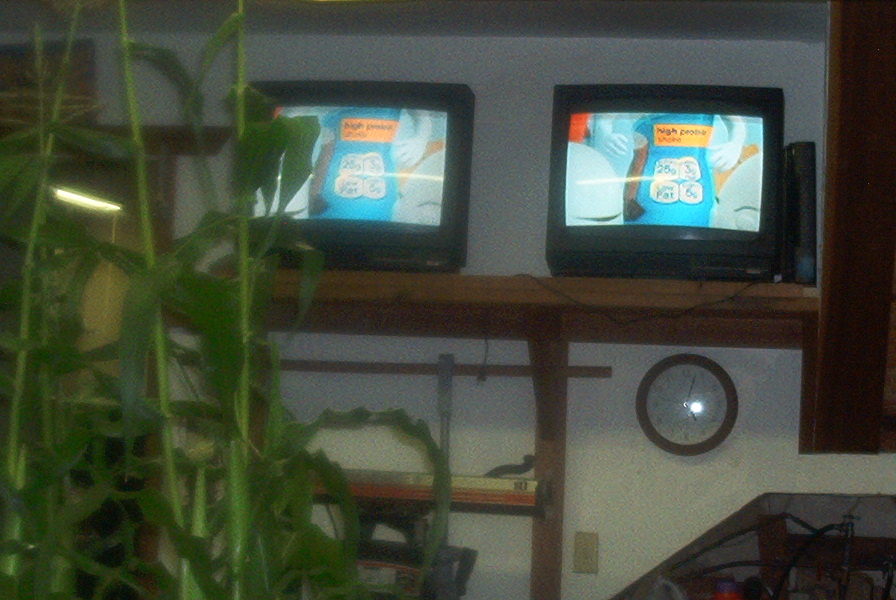This blurry photograph captures a cluttered and eclectic room whose purpose is ambiguous, possibly a garage, basement, storeroom, or waiting area. Dominating the left side of the frame is a tall, green, house plant with large, spiky stalks and dark green leaves. In the background, partially obscured by the plant, is a narrow doorway revealing a long, hospital-like, fluorescent light.

Central to the image are two old-style tube televisions, approximately 19 to 21 inches each, placed on a high, brown wooden shelf mounted on a white wall. Both TVs are tuned to the same channel, displaying a scene featuring a lady in a blue dress with white gloves, along with a yellow banner of some sort, possibly an advertisement mentioning "whey" and "low fat," though it’s unclear due to the blurriness.

Beneath the televisions sits a white-faced, round clock encircled by a brown wooden rim. Supporting the high shelf are brown wooden brackets, and beneath it, scattered objects and an electrical socket can be seen. To the bottom right, another piece of wood or a panel, possibly housing electrical components, adds to the chaotic feel. Overall, the room's contents and poor lighting contribute to a sense of disorganization and mystery.